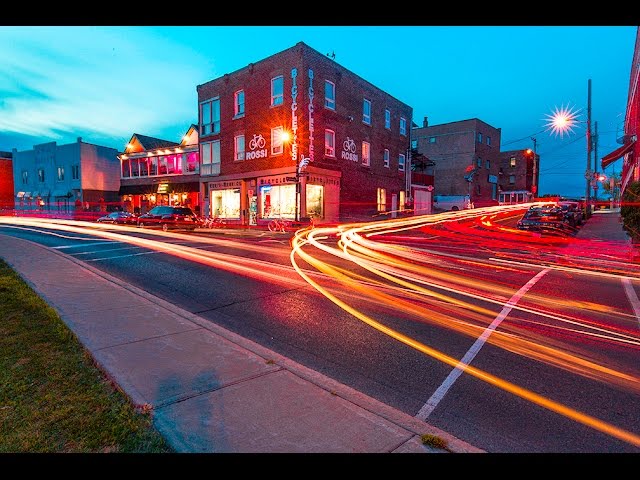The photograph is a captivating night-time cityscape, likely taken with a long exposure or time-lapse technique. The sky is a dark blue, revealing the remnants of daylight as the sun sets. Prominently featured is an intersection where vibrant ribbons of light from car headlights and taillights streak in multiple directions, vividly illustrating the movement and energy of the scene. These light trails intertwine at the crossing, suggesting a busy two-way street.

In the foreground, the viewer's perspective appears to originate from a grassy area adjacent to a sidewalk, giving a grounded point of view. The street is flanked by several buildings, most notable among them being the Rossi Bicycle Tires shop, a brick establishment that stands out with illuminated windows and a clearly visible sign. The presence of streetlights and the subtle glow of a bright object that could be the moon on the right-hand side further enhance the nighttime atmosphere. Despite the night setting, the busy activity of vehicles and the illuminated surroundings invoke a lively small-town charm.